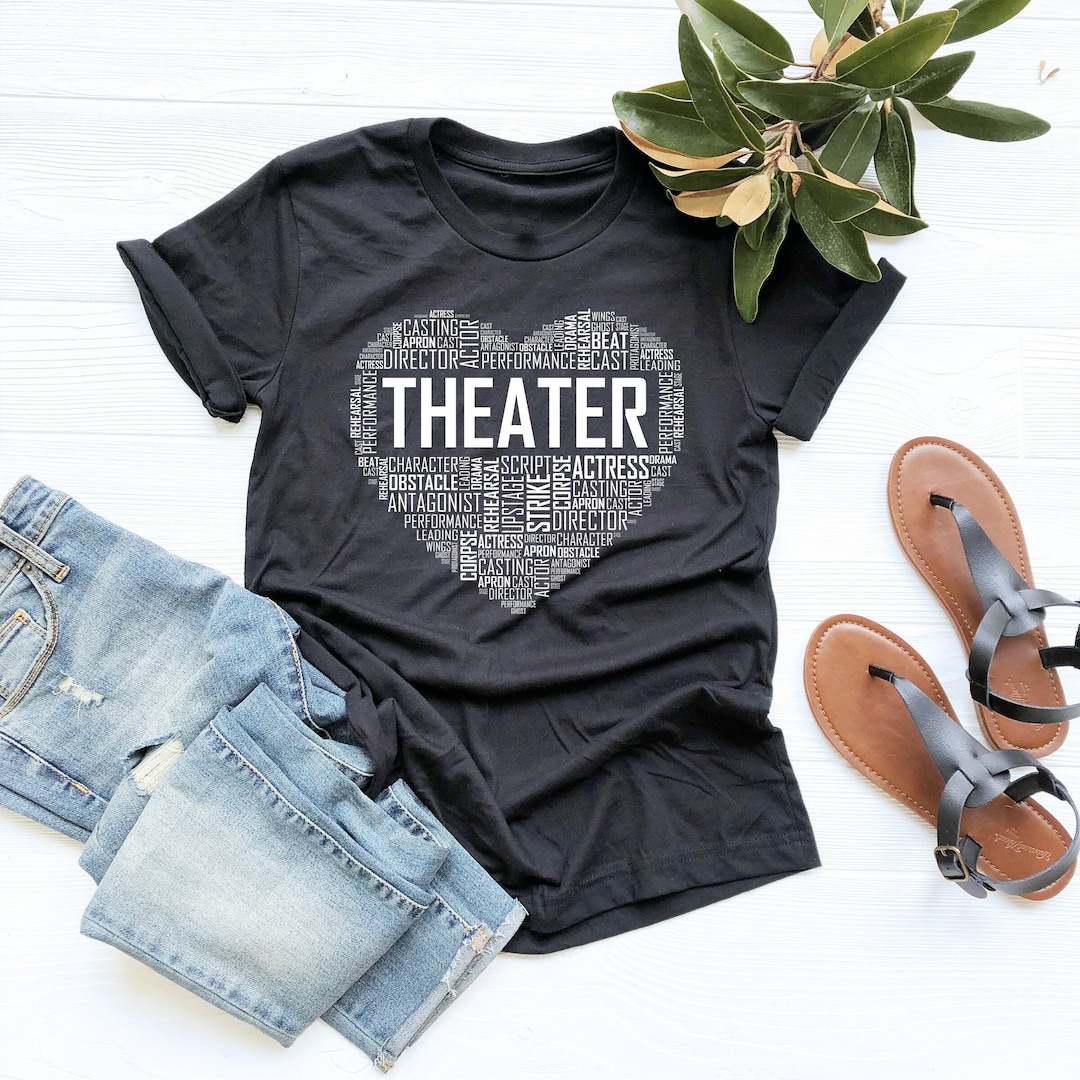This advertising image features a meticulously staged outfit against a backdrop of white faux wood slats. At the center of the photograph is a dark gray, almost black, short-sleeved t-shirt with rolled-up sleeves. The t-shirt prominently displays a large white heart design composed of various theater-related words such as "director," "performance," "character," and "casting," arranged in different directions. The word "THEATER" is boldly highlighted in white, uppercase letters in the center of the heart.

To complement the t-shirt, a pair of lightly washed jeans is neatly folded and placed to the left, partly overlaying the shirt. The jeans are folded lengthwise and then accordioned, emphasizing the casual, ready-to-wear nature of the outfit. To the right of the t-shirt, there is a pair of simple brown and black sandals, adding a practical and stylish touch to the ensemble. Over the top right corner of the image, extending over the shoulder of the t-shirt, is a vibrant leafy branch, adding a natural and fresh element to the presentation.